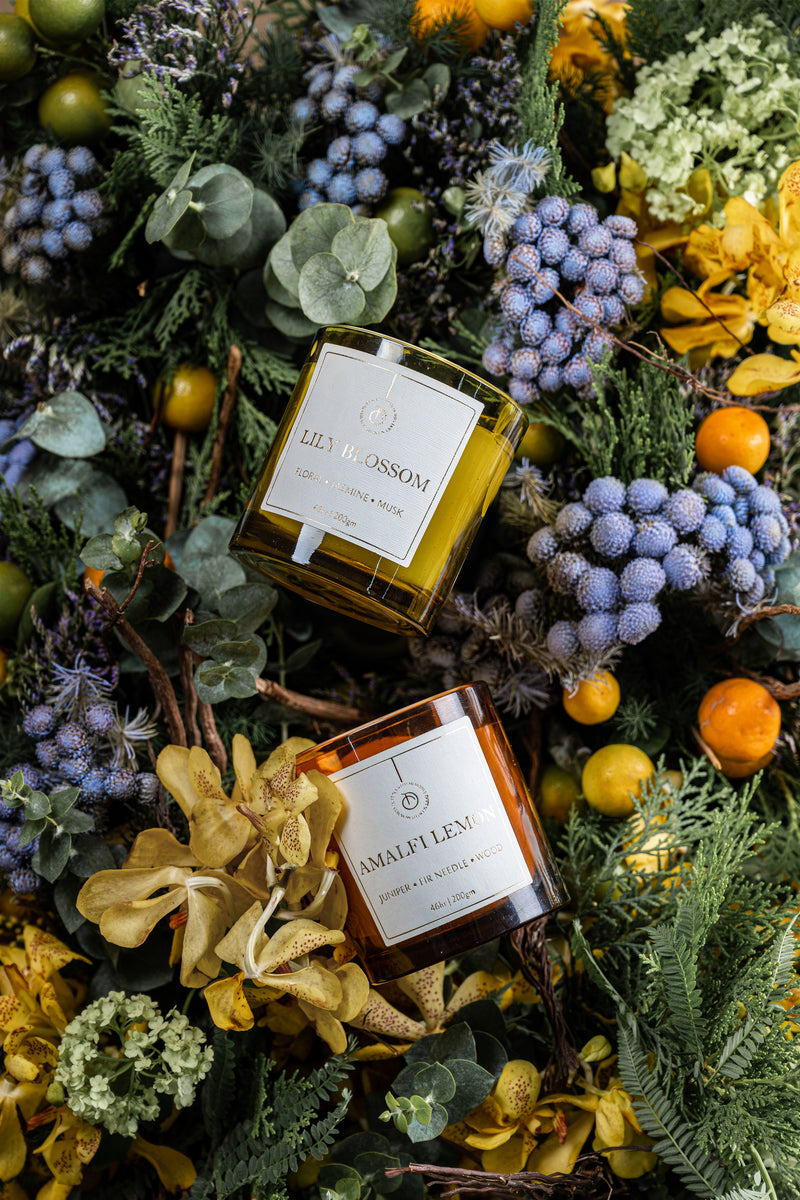This is a detailed, colored indoor photograph showcasing two elegant scented candles set on a lush, intricate bed of botanical elements. The candles are encased in glass jars with distinctive colors; the top candle, labeled "Lily Blossom" in gold metallic letters on an off-white label, rests in a yellow-tinted glass jar. The wax within seems to match the yellow hue of the jar. The lower candle, labeled "Amalfi Lemon," has an off-white label with gold text and is housed in an orange-tinted glass jar with similarly colored wax inside. These candles are nestled among a rich assortment of dried flowers, including frosted grapes, eucalyptus leaves, purple dried flowers, sprigs of fern and spruce, and pieces of citrus fruits such as lemons and orange tangerines. Adding to the festive and luxurious feel, the arrangement includes golden ribbons and bows. Despite the dense foliage and various decorations suggesting a Christmas-themed setting, the primary focus remains on the elegantly displayed candles, likely intended for a promotional advertisement.